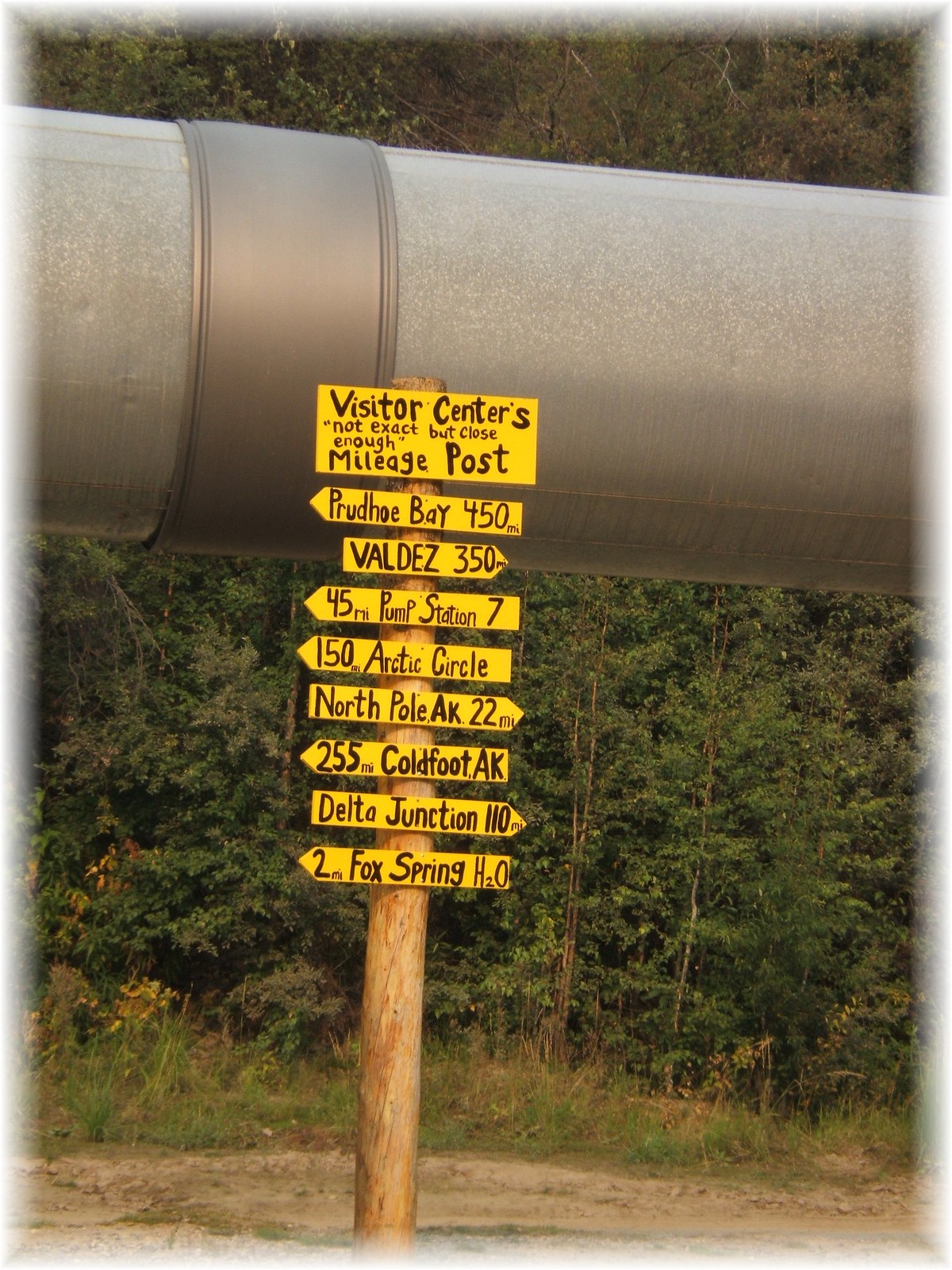The image features a sign resembling a weathervane mounted on a thick wooden pole, situated in front of a backdrop of dense trees, suggesting a location near a hiking trail or natural area. The sign, composed of nine bright yellow miniature signs with black text, provides directional information and distances. The topmost sign reads, "Visitor's Center. Not exact, but close enough mileage post." Below it, the signs point in various directions with the following details:

- Prudhoe Bay: 450 miles to the left
- Valdez: 350 miles to the right
- Pump Station 7: 45 miles to the left
- Arctic Circle: 150 miles to the left
- North Pole, AK: 22 miles to the right
- Coldfoot, AK: 255 miles to the left
- Delta Junction: 110 miles to the right
- Fox Spring H2O: 2 miles to the left

A large pipe, possibly part of industrial infrastructure, runs horizontally behind the sign, blending into the natural setting.